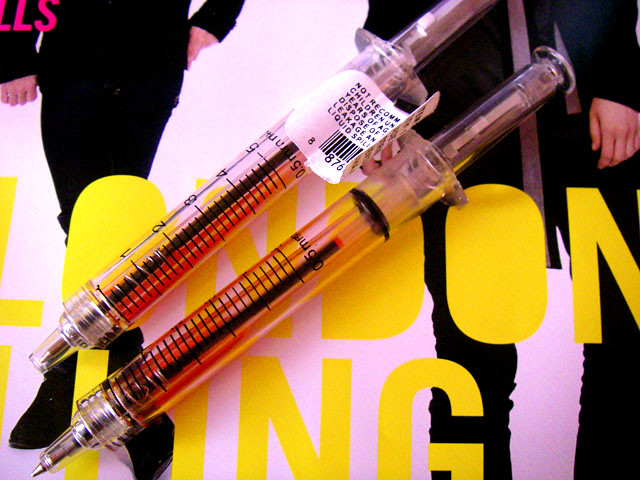This image depicts a close-up view of two clear syringes that have been transformed into ballpoint pens, positioned atop a white advertisement poster. The syringes-turned-pens, which retain their original measurement markings from one to five, now contain dark-colored ink sticks instead of needles. Each pen features inscriptions and warning labels—one specifically displaying a barcode and cautionary text about potential leakage and being not recommended for children. In the background, the advertisement showcases elements of a digital photograph with distinct design features, including purple letters 'LLS' in the upper left corner and the partially obscured word 'London', with filled-in 'O's and 'D'. The ad appears to market clothing, featuring two figures dressed in head-to-toe black, though only their hands are visible. The syringes are slanted, with the pen tips pointed downward toward the lower left corner of the image.